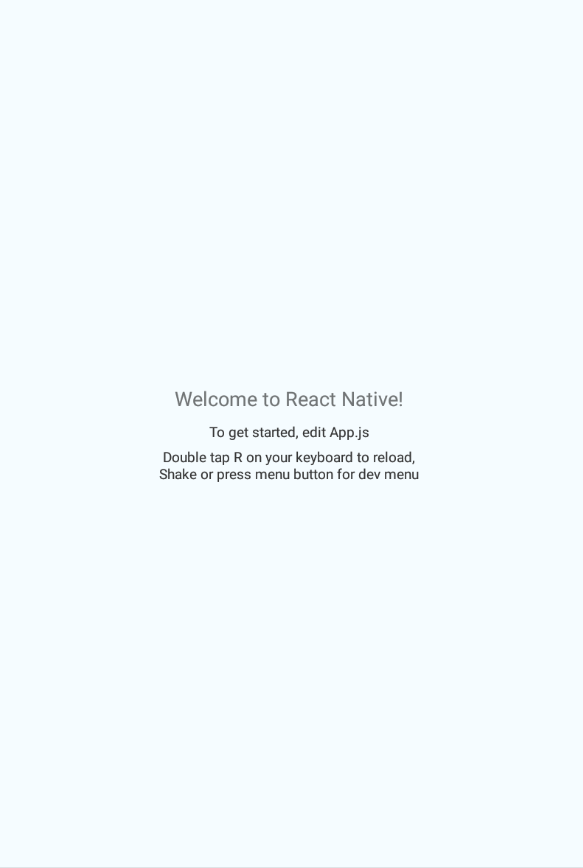The image showcases a minimalistic and clean interface with a background that transitions subtly between light blue and white. Dominating the center of the image is the text "Welcome to React Native!" displayed in a medium-sized, gray font. Beneath this primary message, smaller black text provides guidance for new users: "To get started, edit App.js." Further instructions follow in even smaller font, "Double tap R on your keyboard to reload," and "Shake or press menu button for dev menu." The visual composition is predominantly vertical, with all text neatly aligned in the middle. No photographs or decorative elements distract from the instructional content, emphasizing the simplicity and clarity of the initial setup screen in a React Native environment.